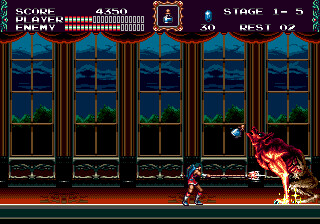The image is a screenshot from an older video game, likely reminiscent of eras such as the Sega Genesis. Set within what seems to be an opulent mansion, the environment showcases elaborate gold and burgundy drapery hanging from five large, ornately designed windows, with glimpses of dark blue clouds and green shrubbery visible outside. The mansion's ceiling towers high, suggesting a grand scale.

In the game, a female character clad in a gladiator outfit, with a shield on her back and boots, holds an electrified sword. She is depicted in battle against a towering, red-and-yellow wolf-like monster, which appears to be about four times her size. At the top of the screen, a HUD displays "SCORE: 4,350" on the left, followed by "PLAYER" with a corresponding health meter, and "ENEMY" with a more full health meter. In the center of the top banner, there is an image that looks like a bottle, alongside a gemstone icon with the number "30" beneath it. To the far right, it reads "Stage 1 to 5, Rest 02". The scene is set on a large red floor, adding to the luxurious feel of the mansion backdrop.